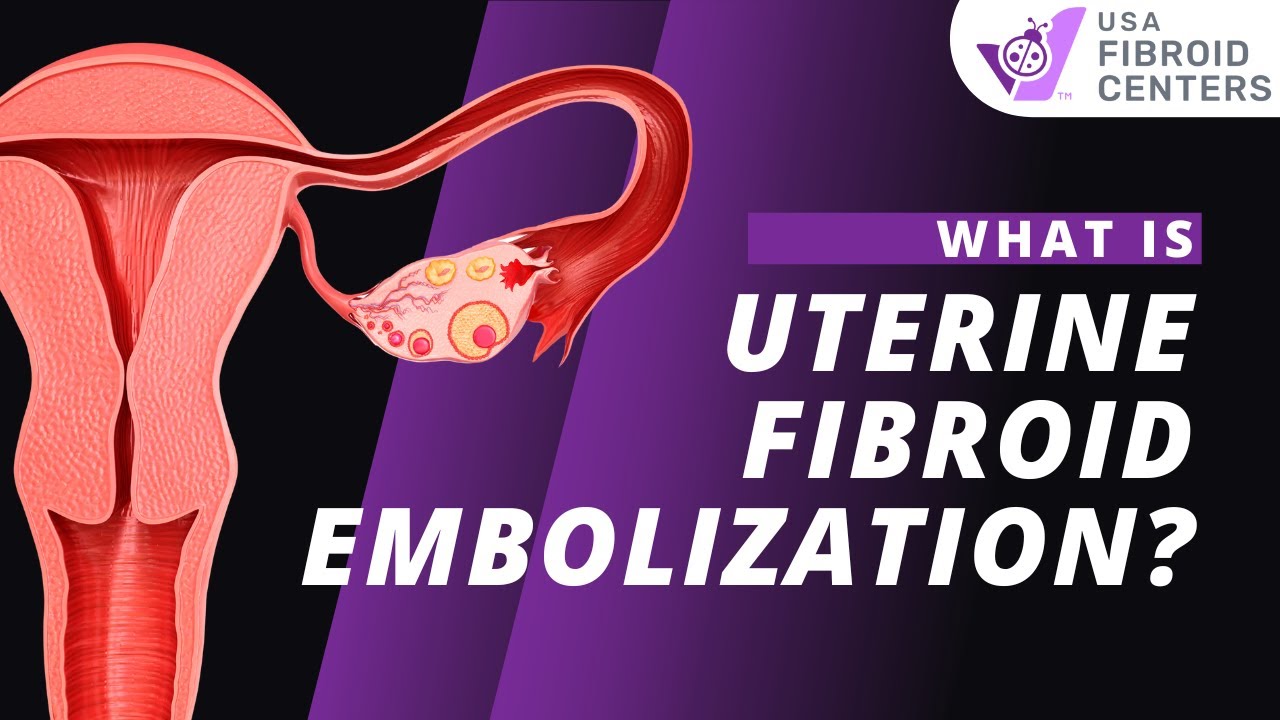This image, related to the USA Fibroid Centers, features a prominently placed logo in the top right corner—a small ladybug atop a purple checkmark accompanied by the trademark designation (TM). The logo sits on a background blending black and purple. The main focus of the image is on the left side, displaying a detailed anatomical illustration of the female reproductive system in shades of red and pink. The anatomical depiction includes the uterus, fallopian tubes, ovaries, and cervix, with visible fibroids indicated in the uterus. The background behind this illustration transitions from black to purple using gradient stripes extending towards the right. To the right of the anatomical image, bold white text on a purple rectangle poses the question: "What is uterine fibroid embolization?" This visualization creates a balanced composition, accentuating the medical focus on uterine fibroid embolization while maintaining a cohesive color scheme throughout the graphic.